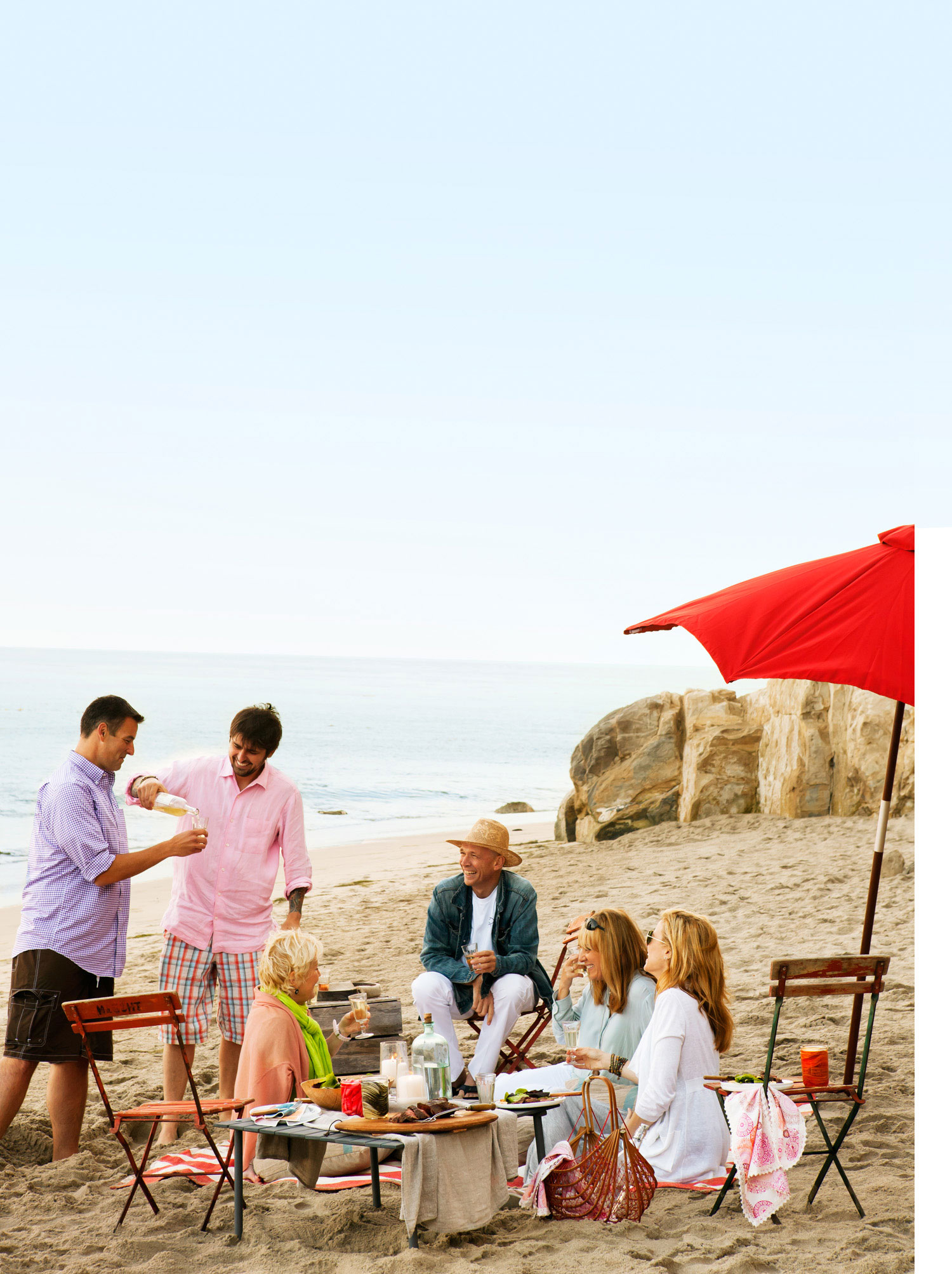The image captures a vibrant beach scene on a clear, sunny day with a striking blue sky devoid of clouds. The foreground is centered around a lively group of six people enjoying a beach picnic. Seated around a table, adorned with red cups and food, are three women and three men, all seemingly in their 30s to 40s. On the left, under a red umbrella, the three women are seated on the sand, not on the small chairs around them. The woman on the far left sports a peach-colored shirt with a green scarf, while the other two women wear white tops.

In the middle of the group, an older man in a hat, a blue coat, and white pants appears relaxed and content. To the left, two men stand; one, in a pink dress shirt and plaid shorts, pours a drink for the other, who wears a light purple (or blue) dress shirt paired with dark blue shorts. Their dark hair and casual demeanor suggest they are possibly in their 30s or 40s as well.

The background features a picturesque stretch of blue ocean and a light brown rock, adding a tranquil and scenic touch to the lively foreground. The entire scene suggests a leisurely, joyful beach gathering, with beachgoers enjoying food, drinks, and each other’s company beside the gently crashing waves and warm, sandy shore.